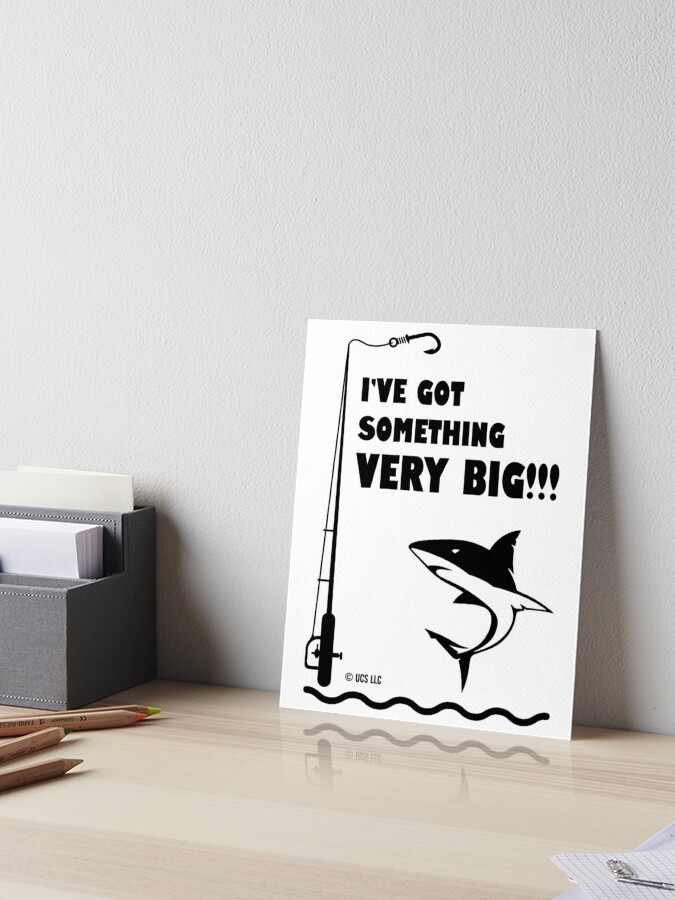This is an image of a pale wooden desk pushed against a light gray wall in an indoor setting with natural light. The desk is organized with various office supplies. On the left side, there is a gray organizer holding envelopes and stationery, with three visible colored pencils—a lime green, orange, and black—positioned in front. Additionally, there are plain wooden pencils on the bottom left, and a lined piece of paper with paperclips on the bottom right. 

The most prominent feature is a white cardstock poster leaning against the wall, measuring roughly 6 by 8 inches. It features a simple black line drawing: a fishing pole on the left extending the full height of the card, with a string and hook over the words. The bold, block-lettered text reads, "I'VE GOT SOMETHING VERY BIG!!!" with three exclamation points. Below the text is an illustrated shark with a black upper body and a white underside, appearing to leap out of stylized wavy water lines at the bottom. The entire drawing is in black and white, and there's an indistinct copyright mark at the bottom.